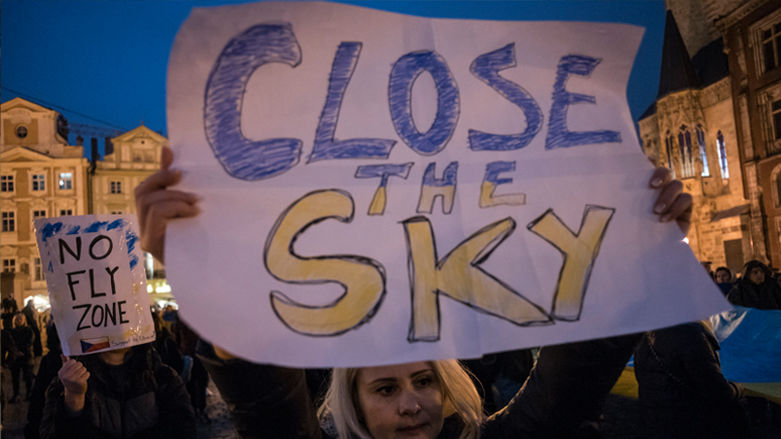The image depicts a protest occurring in the early evening, either just at or just past dusk. The central figure is a blonde-haired woman prominently holding a sizeable, handmade sign that reads "Close the Sky." The sign is crafted on a substantial white piece of paper with "Close" written in blue, "the" directly below in smaller text, with the top half of the letters in blue and the bottom half in yellow, and "Sky" written entirely in yellow. These colors represent the Ukrainian flag. Surrounding her is a crowd of people, some carrying Ukrainian flags. To her right, another individual holds a smaller sign that reads "No Fly Zone." The gathering is taking place on a street with visible buildings in the background, which are faintly illuminated by streetlights. The sky above is darkening, indicative of evening time.